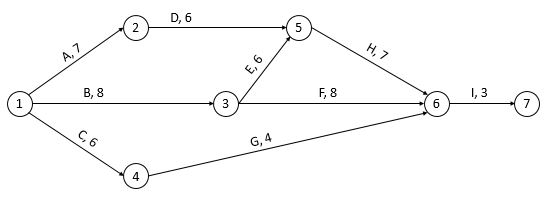This image features a simple, hand-drawn diagram on a plain white piece of paper. The diagram is composed of multiple straight lines intersecting and forming various geometric shapes and pathways. A prominent horizontal line stretches across the entire width of the paper, from left to right. Superimposed over this horizontal line is an outline of a diamond shape, with its edges clearly intersecting the central line.

Interspersed throughout the diagram are a series of numbers and letters. Notably, the numbers 1 and 2 are encased in black circles, while the letter and number combinations such as A7 and D6 appear in between numbered points. Specifically, A7 is positioned between numbers 1 and 2, while D6 lies between numbers 2 and 5. A line descends from the number 5 to the number 3, with E6 marked along this path.

While the purpose of the diagram is unclear, it seems to be a geometric exercise or a schematic illustration, as the lines and points are meticulously labeled but do not form any recognizable real-world object. The drawing appears to be an abstract arrangement of straight lines connected in a methodical, yet puzzling sequence.